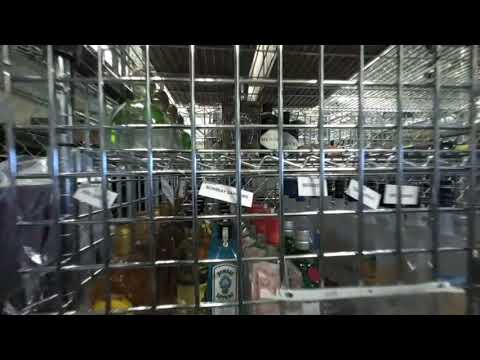The image showcases an indoor setting where various alcohol bottles are secured behind a thick, silver-colored grid of intersecting steel rods forming a cage. The layout of the photograph is framed by thick black rectangles at the top and bottom, giving it a wide rectangular appearance. Central to the composition are several bottles arranged methodically:

1. At the bottom, a prominent blue bottle with a transparent body features a white label and additional white labels with unreadable black text. Adjacent to this, there is a bottle with a pink label and a red cap.
2. Toward the left, a row of brown bottles with yellow labels extends back into the depth of the image.
3. Further right, blue square-shaped bottles with white stickers and black text are prominently displayed.
4. At the far right, green bottles are found, some of which are topped with either red or silver caps, with a notable green goblet-shaped bottle positioned on the top row, extending towards the back.

The top center of the image appears dark while the sides shift to a silver hue. Various colored tags, although unreadable, are positioned centrally in the foreground. The overall palette in the image includes black, gray, silver, blue, red, yellow, orange, and green, emphasizing the diverse assortment of bottles. The heavy steel cage dominates the entire photograph, suggesting a secure storage possibly within a supermarket or shipping container environment, and a light source is visible towards the top.